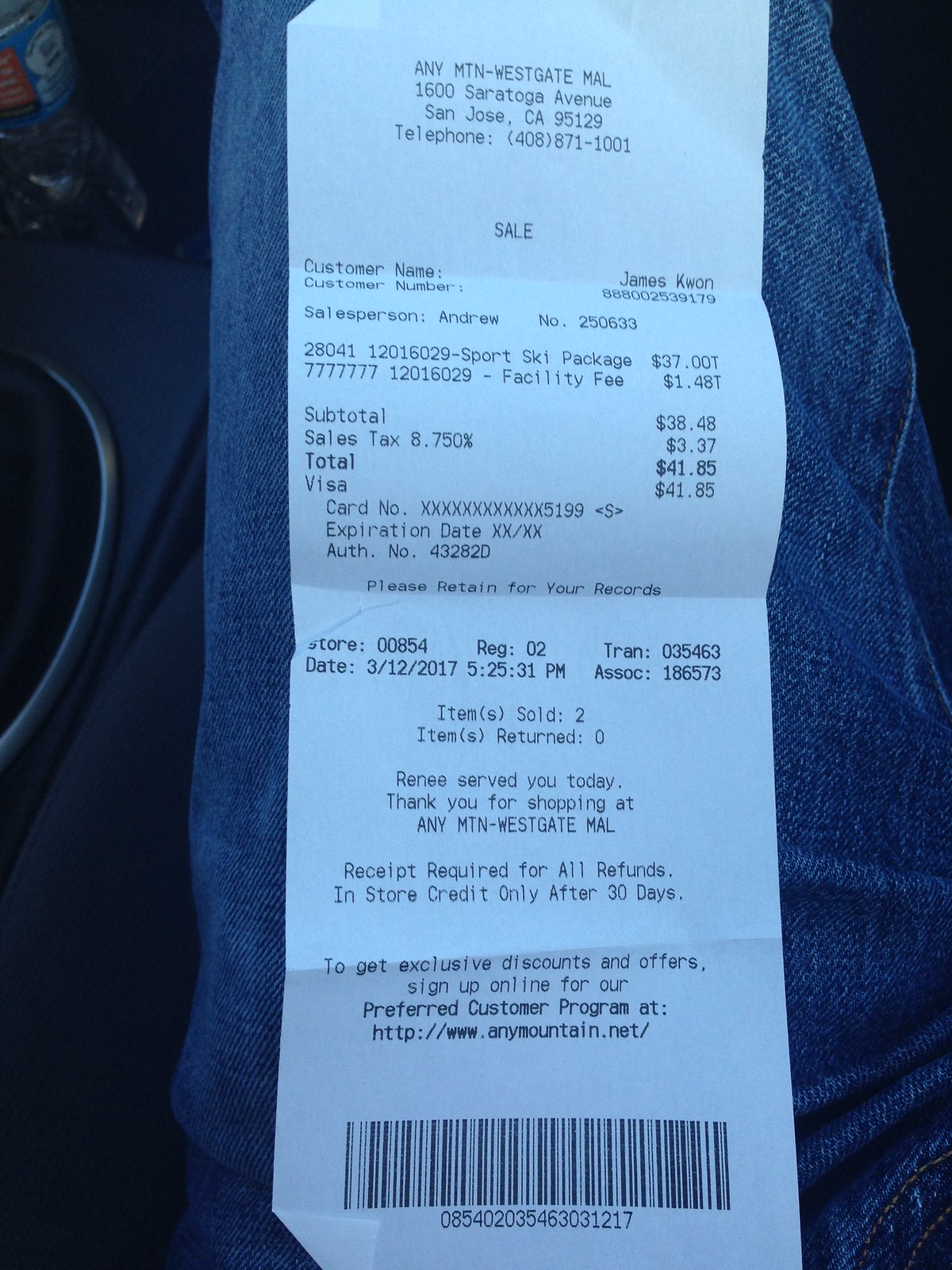A photograph capturing a detailed image of a white paper receipt placed against someone's leg clad in denim jeans. The setting appears to be inside a car, as evidenced by glimpses of a cup holder, a water bottle, and what seems to be the edge of an emergency brake or transmission shifter visible on the left side of the frame. The receipt itself, tall and folded multiple times with visible crease lines, prominently displays "Any Mountain Westgate Mall, 1600 Saratoga Avenue, San Jose, California, 95129" at the top. The purchase listed includes a "sport ski package" and a "facility fee," culminating in a total charge of $4185, with a barcode placed towards the bottom of the receipt.